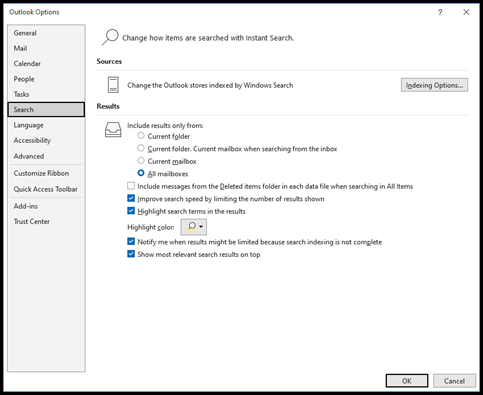The image depicts an Outlook Options web page interface. At the top, a subtle, unbolded heading reads "Outlook Options". Directly below, there's a navigation pane with various sections including General, Mail, Calendar, People, Tasks, and notably, Search, which has been selected by the user, highlighting its relevance to search functionalities.

Several other options are visible in the same font style, including Language, Accessibility, Advanced, Customized Ribbon, Quick Access Toolbar, Add-ins, and Trust Center. The page is focused on the search configuration settings of Microsoft Outlook. Specifically, it provides options related to "Instant Search", hinting at a recent upgrade or customization feature.

The page details ways to change how items are searched using Instant Search. Among these options, it includes a section labeled "Sources," which allows users to alter how Outlook stores are indexed by Windows Search. A button labeled "Indexing Options" is available for further customization.

Under this section, there is a configuration for search results, offering several choices like "Include results only from current folder," "Current Folder," "Current Mailbox," and "All Mailboxes." Finally, at the bottom of the page, users have the option to either finalize their changes by clicking "OK" or discard them by selecting "Cancel."